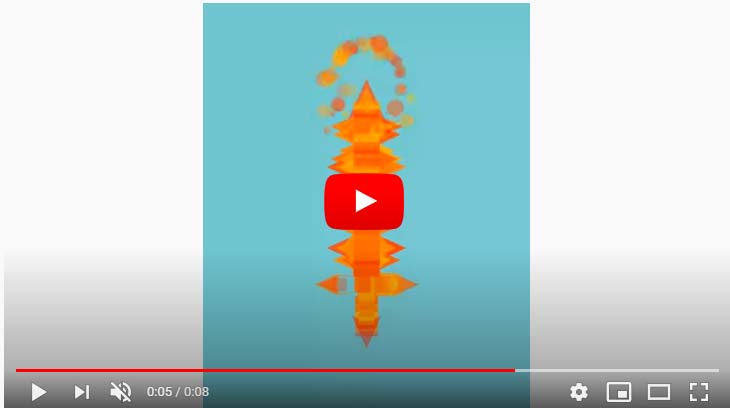The image is a screenshot of a YouTube video paused at 05 seconds out of an 08-second duration, indicated by the red seek bar at the bottom. The quintessential YouTube play button, a red triangle, is prominently displayed in the center overlaid with the YouTube logo, suggesting the video is paused and ready to be played again. 

The video's background features a blue rectangular shape at the center, bordered by white to gray gradients on the sides that transition to black at the bottom edge. Within this blue central area, there are abstract shapes including reddish-orange and fiery blobs, along with green and orange elements, which are flat illustrations. These shapes might be random animations, with some resembling ornamented sticks with small arrows pointing outwards and colored bubbles emerging from the top. 

On the lower portion of the screen, typical YouTube interface elements are visible: the play button, skip button (a triangle with a line), and a muted speech button (a speaker crossed out). Additionally, the lower right includes settings, mini player, theater mode, and maximize buttons, making the YouTube video's user interface distinctly recognizable.